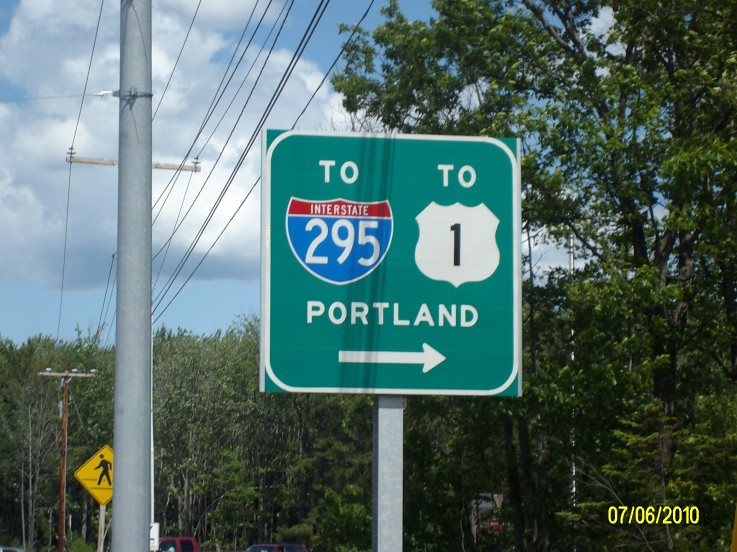A close-up photograph captures a real-life road sign prominently centered in the image. The sign is mounted on a metal post that emerges from the bottom of the frame, its base unseen. Dominating the sign is a green rectangular panel with sharp edges, bordered by a white outline with distinct rounded corners. The green panel features multiple symbols and text: a large white number "2," a blue and red shield symbol indicating "Interstate 295," and a smaller white shield symbol with a black number "1." Above the smaller shield, another white number "2" is depicted. Below these, the word "Portland" is written in white with a rightward-pointing arrow.

In the background, a dense forest of countless trees forms a natural backdrop. To the left of the road sign stands a towering metal pole, likely an electric utility pole, extending out of the frame and carrying multiple electrical wires. Further left and slightly back, an additional wooden utility pole supports the same set of wires.

Behind the electric pole, another road sign, this one diamond-shaped and yellow with a black border, stands visible. This secondary sign bears a black icon of a person crossing the road.

At the bottom right of the image, a digital timestamp in yellow numerals reads "07/06/2010," indicating the date the photograph was taken.